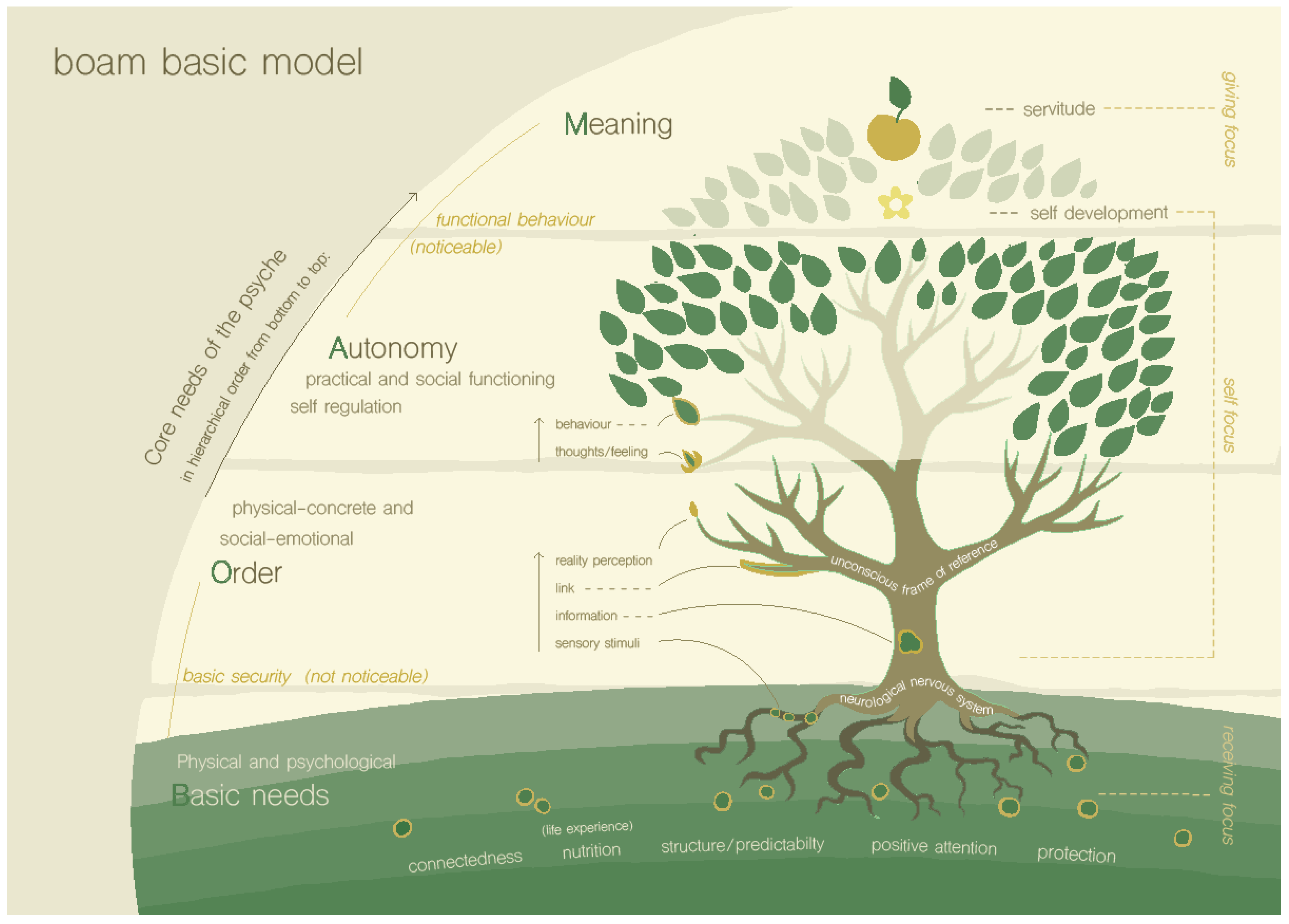This image is a detailed diagram illustrating the core psychological needs of a person using a tree metaphor, intended for a book or poster. At the top left corner of the diagram, it is labeled "BOAN Basic Model," and the phrase "Core Needs of the Psyche, in hierarchical order from bottom to top" is inscribed along the left side. 

At the base of the image, the ground is covered in various shades of green. Below ground, the roots of the tree are labeled "Physical and Psychological Basic Needs," including elements such as Connectedness, Nutrition, Attention, and Protection, and are connected to the "Neurological Nervous System."

Above ground, the diagram is split into three sections, all in an off-white color. The tree trunk, rising just above the ground, represents Sensory Stimuli, Reality Perception, and Social Information Link. As the trunk branches out, the sections marked include "Physical Concrete," "Social Emotional Order," and "Autonomy Practical and Social Functioning." 

Further up, where the tree's branches are more spread out and the leaves are larger, the sections are labeled "Self-Regulation," encompassing behavior, thoughts, and feelings. A bracket titled "Self-Focus and Self-Development" is indicated on the right side. Finally, at the very top, where the tree is full and rounded, it reads "Functional Behavior" and is marked by self-development and servitude, signifying the attainment of meaning in one's life.